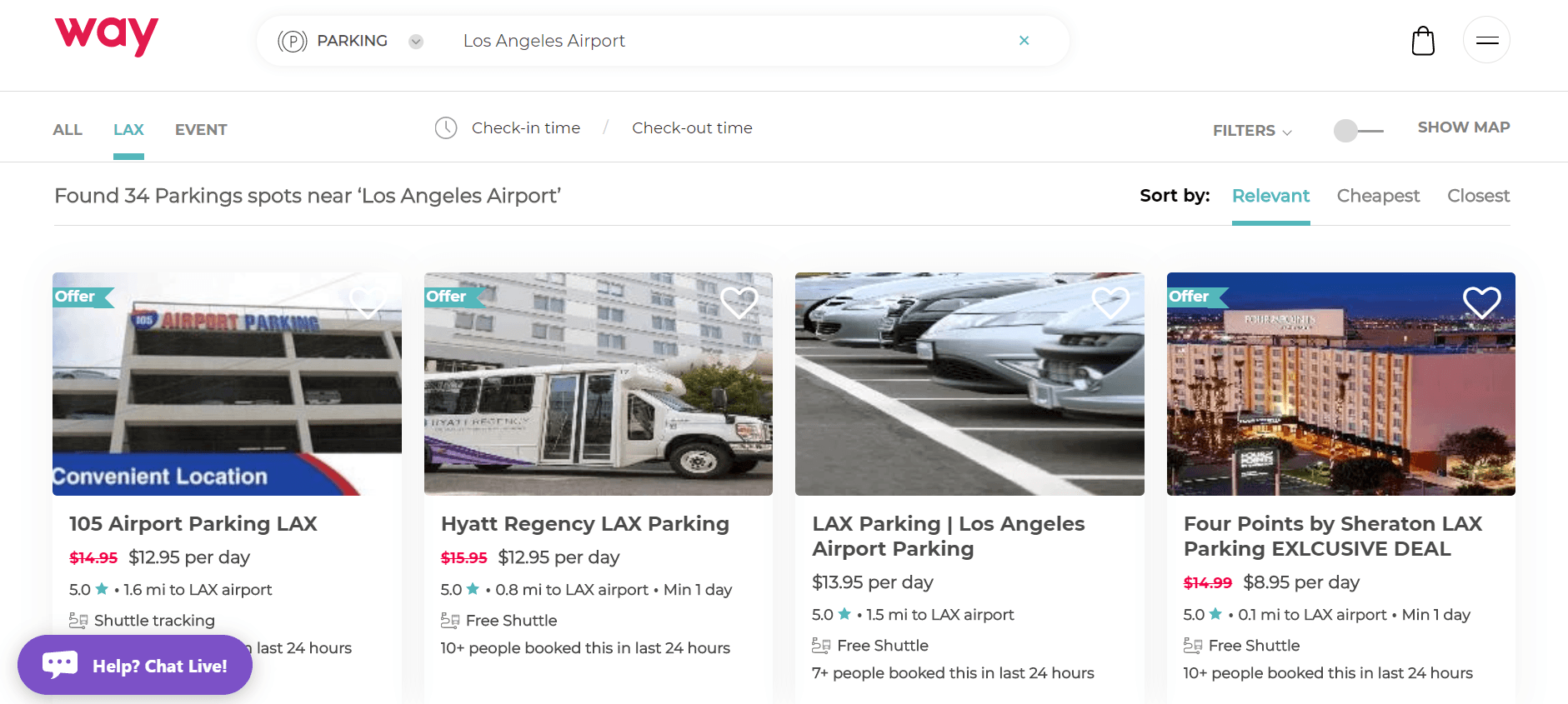The image depicts a webpage thumbnail from a website named "Way," with its logo positioned in the top left corner in red font. Adjacent to the logo, there is a text box drop-down menu, currently displaying "Parking," with "Los Angeles Airport" typed in the search field. This is central and slightly to the left. Icon elements and two additional menu items align to the right on the same top row. 

Beneath this, there is a secondary navigation bar featuring options such as "All," "LAX," and "Event," with "LAX" currently selected. Further to the right on this bar, sections for entering check-in and check-out times, along with filters, are visible but unselected. Below this, the page indicates "Found 34 parking spots near Los Angeles Airport" on the left side of the third line.

Directly below this notice, there is a sorting menu with options like "Relevant," "Cheapest," and "Closest," with "Relevant" highlighted in green. The main section of the page displays four thumbnail images of different parking options near LAX. Each thumbnail is accompanied by pertinent details about the parking spots. At the bottom right corner of the webpage, there is a purple "Help Chat Live" button.